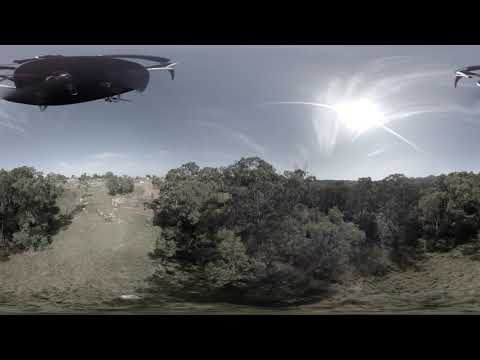The photograph appears to be an outdoor scene, possibly a still from a show or a panoramic image captured by a drone, given its 360-degree quality and slight warping. The sky occupies about half of the image and is predominantly gray with some misty clouds, suggesting the colors have been slightly desaturated. A white helicopter or possibly a drone is visible in the upper left corner, resembling an airplane wing. The landscape below features a wild assortment of shrubs and trees scattered across a patchy ground interspersed with dirt paths. The vegetation is not curated but rather natural and dense, forming two distinct sections with a dirt path running between them. The scene conveys a somewhat distorted view, likely due to the method of capture, adding an intriguing, almost surreal quality to the image.